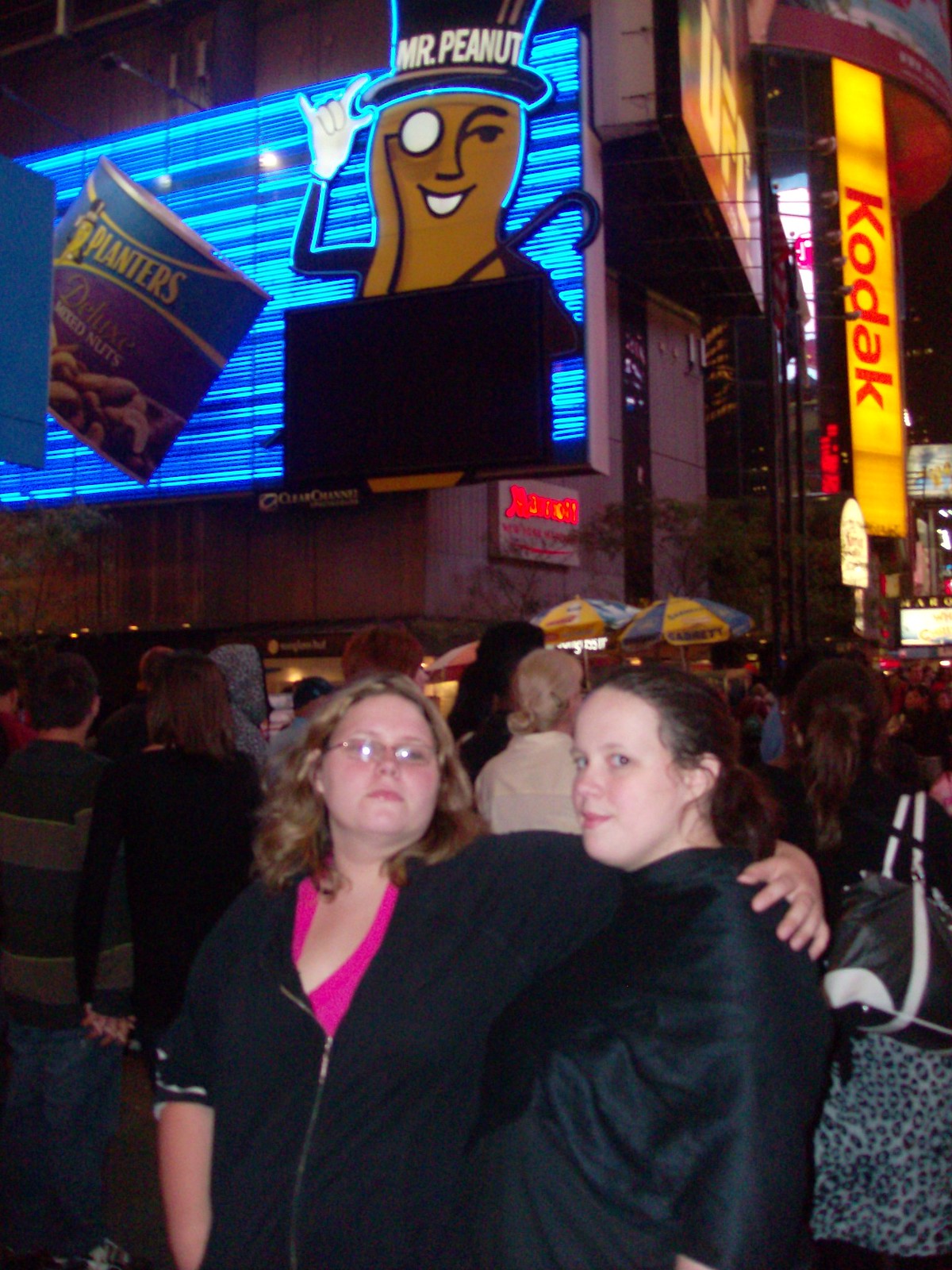This color nighttime photograph captures an energetic city street scene with a dense crowd centered around various illuminated advertisements. Dominating the backdrop is a bright blue electronic display showcasing the iconic Mr. Peanut, a gold anthropomorphic peanut wearing a black top hat with "Mr. Peanut" in white lettering. Beside him is an image of a can of Planters Deluxe Mixed Nuts. To the left, another towering sign features the word "Kodak" in red within a yellow border. The emblem of the Marriott Hotel can also be seen on the building.

In the foreground, two women stand close together, looking directly at the camera. The woman on the left has blonde hair, wears glasses, and is dressed in a black zip-up jacket over a pink shirt. She has her arm around the other woman, who has brown hair and is wearing a black short-sleeve top that reveals a bit of her midriff. Both have fair skin and are posing for the photo.

Surrounding the women is a bustling crowd, most of whom are facing away from the camera. Notably, a man in a green striped shirt holds hands with a woman with long brown hair, both visible on the left. Hot dog stands pepper the scene, enhancing the urban ambiance, suggesting a lively nighttime outing.